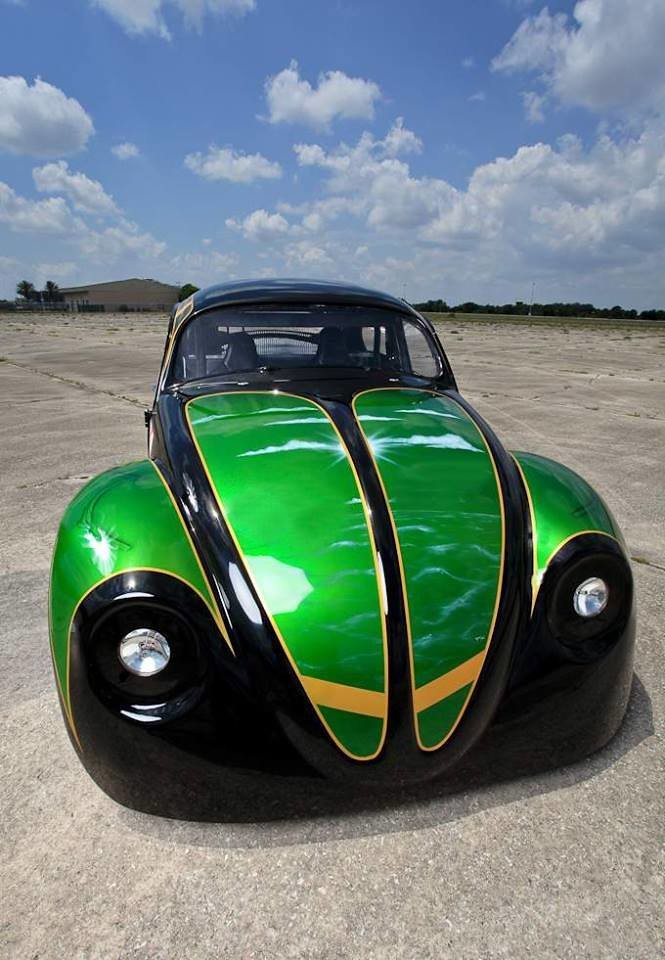In this image, we see a large outdoor concrete area extending to the horizon, where a small strip of grass and some trees are visible on the left side, along with a white-walled building. Above, the sky is partly clouded with sections of open blue sky. The central focus of the image is a unique and striking frontal view of a modified, hot-rodded Volkswagen Beetle. The car features a polished, glossy black exterior with vivid green and golden accents. Around the headlights, green details with golden borders stand out, while the hood boasts two prominent green shapes, also bordered in gold, that taper diagonally. The fenders mix a green metallic hue with yellow borders, and the roof maintains a sleek black finish. The overall reflectiveness and the carefully executed paint job suggest this car is meticulously maintained, likely intended for showrooms or car shows. The design exudes a sense of modern, supercar flair while retaining the classic charm of the Beetle. Only two seats are visible, indicating it is a two-seater model.